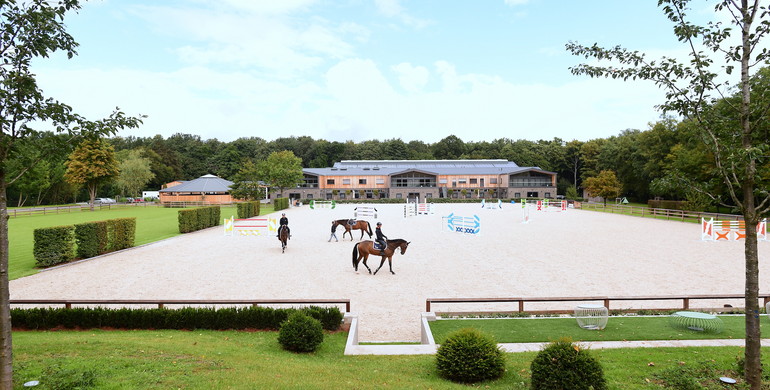In this colorful outdoor photo, we see an extensive equestrian training area. The field, approximately 100 meters long and 50 meters wide, features a dirt surface and various fence-like structures for jumping. Three horses are present: two with riders and one being led on foot. The horses appear to be practicing for a jumping event, navigating the obstacles set up at different heights. In the foreground, a low fence with shrubs encloses a circular training zone. Surrounding the entire area are lush grass and an encompassing forest of trees. At the far end of the field, a prominent pink building spans the length of the equestrian training area, adding a distinct backdrop to the scene.